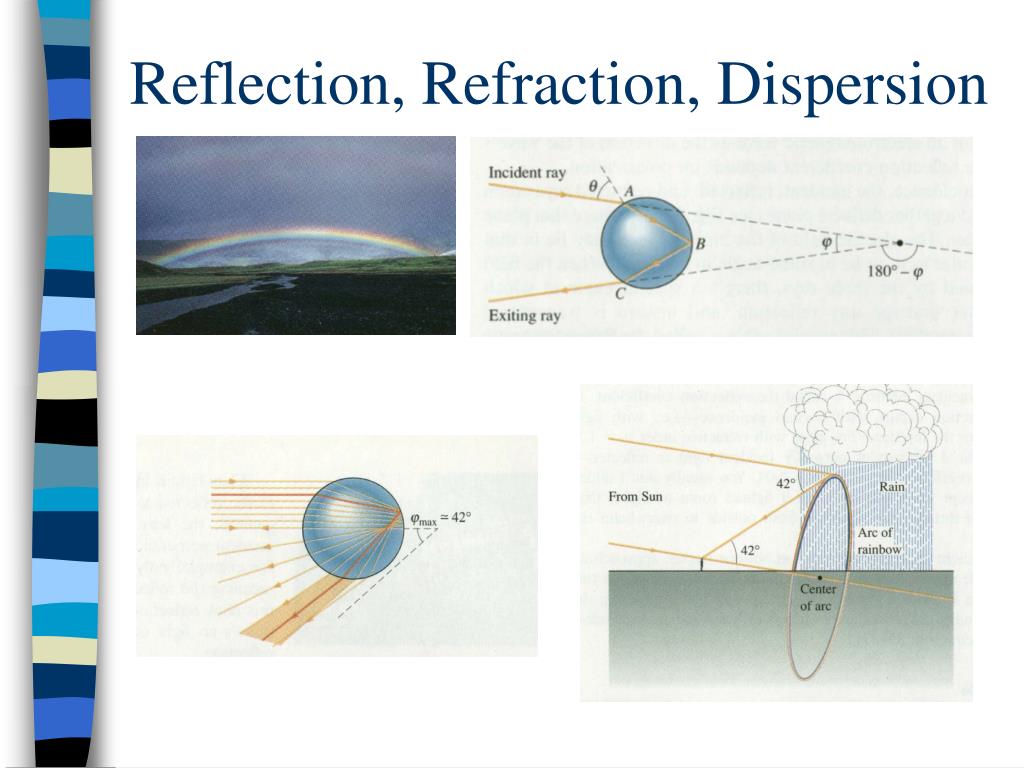The infographic titled "Reflection, Refraction, Dispersion" is prominently displayed at the top in dark blue text. Below this title, the infographic is divided into four panels. The top left panel features a distant, shadowy rainbow set against a dark sky. The top right panel illustrates the principle of refraction with a drawing that includes incident and exiting rays interacting with a blue sphere. The bottom left panel demonstrates reflection, again involving rays and a blue sphere, showing different angles of light interaction. The bottom right panel explains dispersion, depicting an arc that illustrates how a rainbow is formed. The left side of the infographic features a vertical striped border in multicolors, including shades of blue, black, and white, enhancing the visual appeal on a predominantly white background.